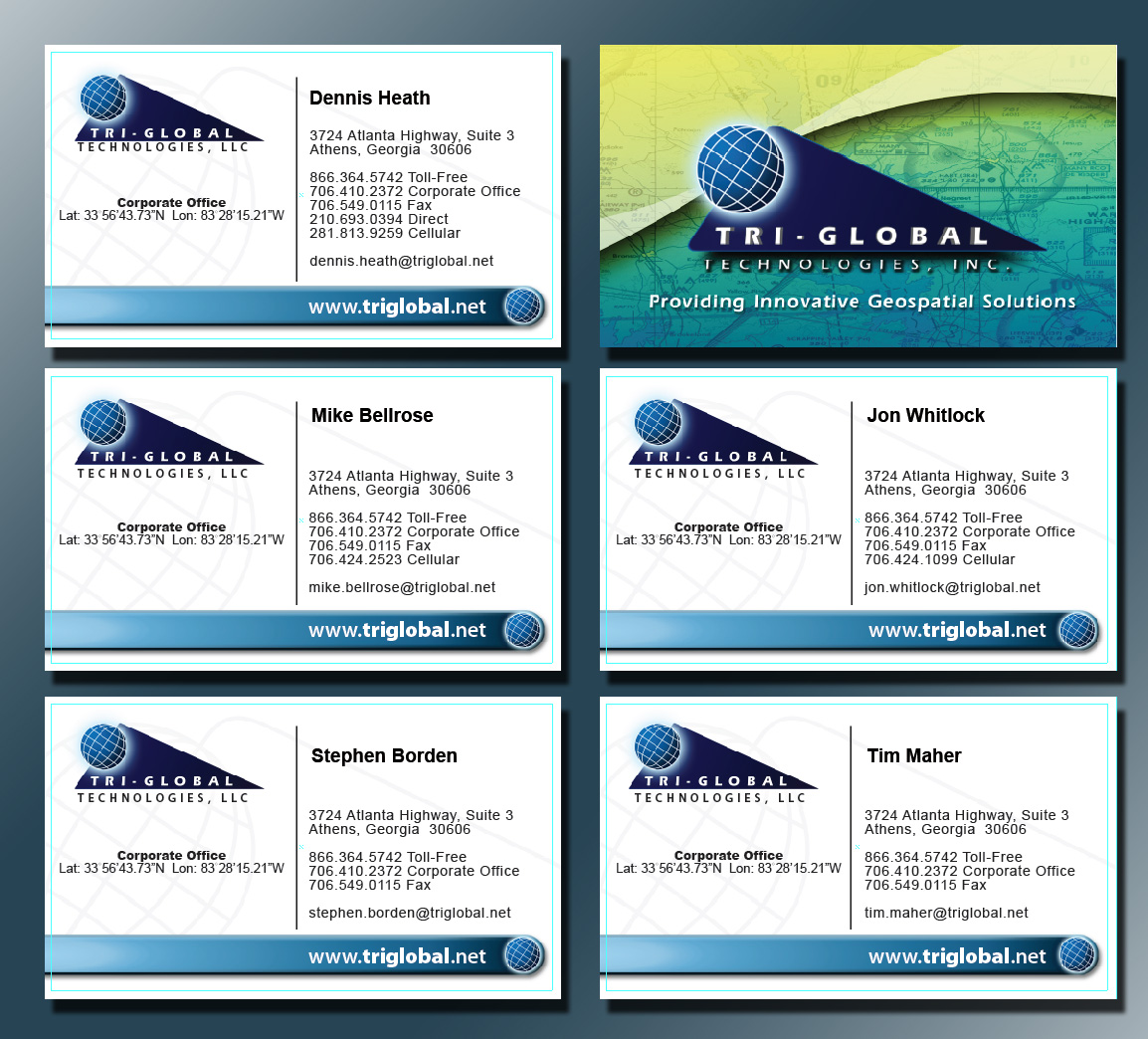The image showcases six identical business cards from "Tri-Global Technologies, LLC," organized in three rows of two. Each business card features a blue globe with a white grid pattern superimposed on a dark blue isosceles triangle that contains the text "Tri-Global" in white block letters and "Technologies, LLC" in smaller black text along the triangle's base. Beneath this, the text "Corporate Office" is displayed above the office's latitude and longitude coordinates. A thin black line runs down the middle of each card, dividing the elements. The right side details the individual's name in black text, followed by their office address, five lines of various phone numbers (toll-free, corporate office, fax, direct, and cellular), and their email address. Highlighted names include Dennis Heath, Mike Belrose, John Whitlock, Tim Meijer, and Stephen Bourdain. The top-right card's reverse side—distinct from the others—displays a larger Tri-Global logo on a blue and yellow gradient map background, with the slogan "Providing Innovative Geospatial Solutions" in white. The uniform office address listed is 3724 Atlanta Highway, Thomas Street 3, Athens, Georgia, 30606.